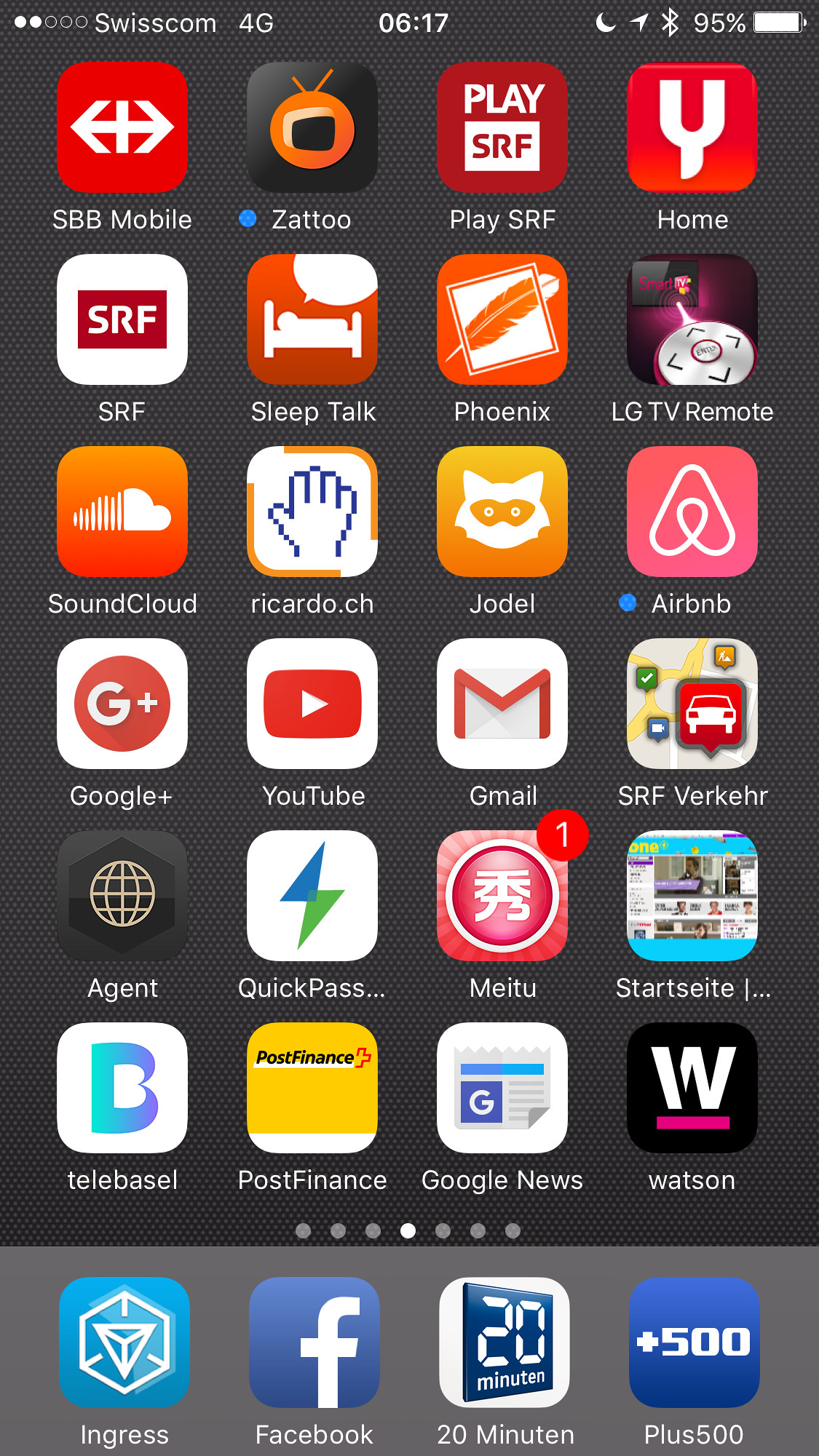The screenshot captures the home screen of an older model smartphone with a 4G connection. The phone, currently at 95% battery life, has Bluetooth enabled, indicated by the icons on the top of the screen. Additional symbols include the moon (likely denoting 'Do Not Disturb' mode) and an arrow. The time displayed is 6:17 without specifying AM or PM. The mobile network reads "4G Swisscom," with only two out of five signal bars filled, suggesting a poor reception.

The background of the home screen is gray, and there are a total of seven pages of apps, as shown by the indicator dots at the bottom. The apps visible in the screenshot include:

1. SBB Mobile
2. Z2
3. Play SRF
4. Home
5. SRF
6. Sleep Talk
7. Phoenix
8. LG TV Remote
9. SoundCloud
10. Ricardo.ch
11. Jodo
12. Airbnb
13. Google Plus
14. YouTube
15. Gmail
16. SRF (again)
17. Verk
18. Her
19. Agent
20. Quick Pass
21. Mate 2
22. Start
23. Site
24. Telebasil
25. PostFinance
26. Google News
27. Watson
28. Ingress
29. Facebook
30. 20 Minuten
31. Plus500

Overall, the detailed depiction highlights the extensive array of applications organized on a cluttered yet functional home screen.